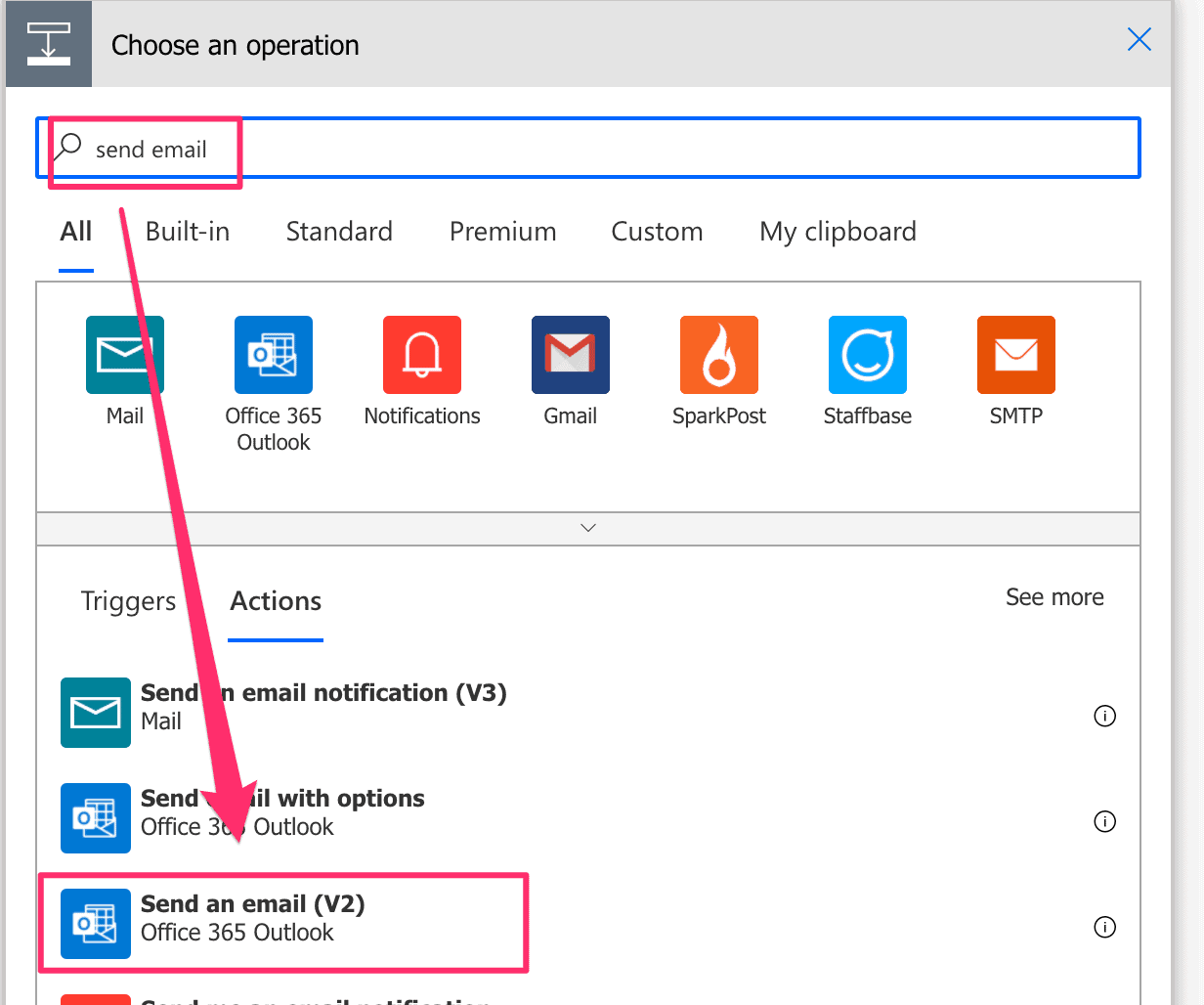In the upper left corner of the image, there is a dark blue square with a white open box icon inside it, which contains a downward arrow and a fully filled white box. Next to this icon, on a bluish-gray background, there is black text that reads "Choose an option." On the right-hand side of this section, there is a gray 'X' icon.

Below this, in another blue square, there is a gray magnifying glass icon accompanied by the text "Send Mail" on the left side. This section is highlighted by a red outline and further emphasized by a pinkish downward-pointing arrow. 

The text "All built in standard, premium, custom clipboards," appears underneath, followed by a list of mail options: "Mail, Outlook 365 Notifications, Gmail, SparkPoint, StaffBase, and SMTP." 

In the next background section, there is text specifying "Triggers and actions," with a "See more" option available. This section lists out options such as "Send email notification V3," "Send mail with options," with a pinkish arrow pointing at "Send Mail V2," which is highlighted with a pinkish color. 

Above the "Triggers and actions" label on the right-hand side, another "See more" option is displayed. The image also features three circles containing an 'i' icon for each previously described option. 

This concludes the description of the current image, which will be followed by reviewing the next one.